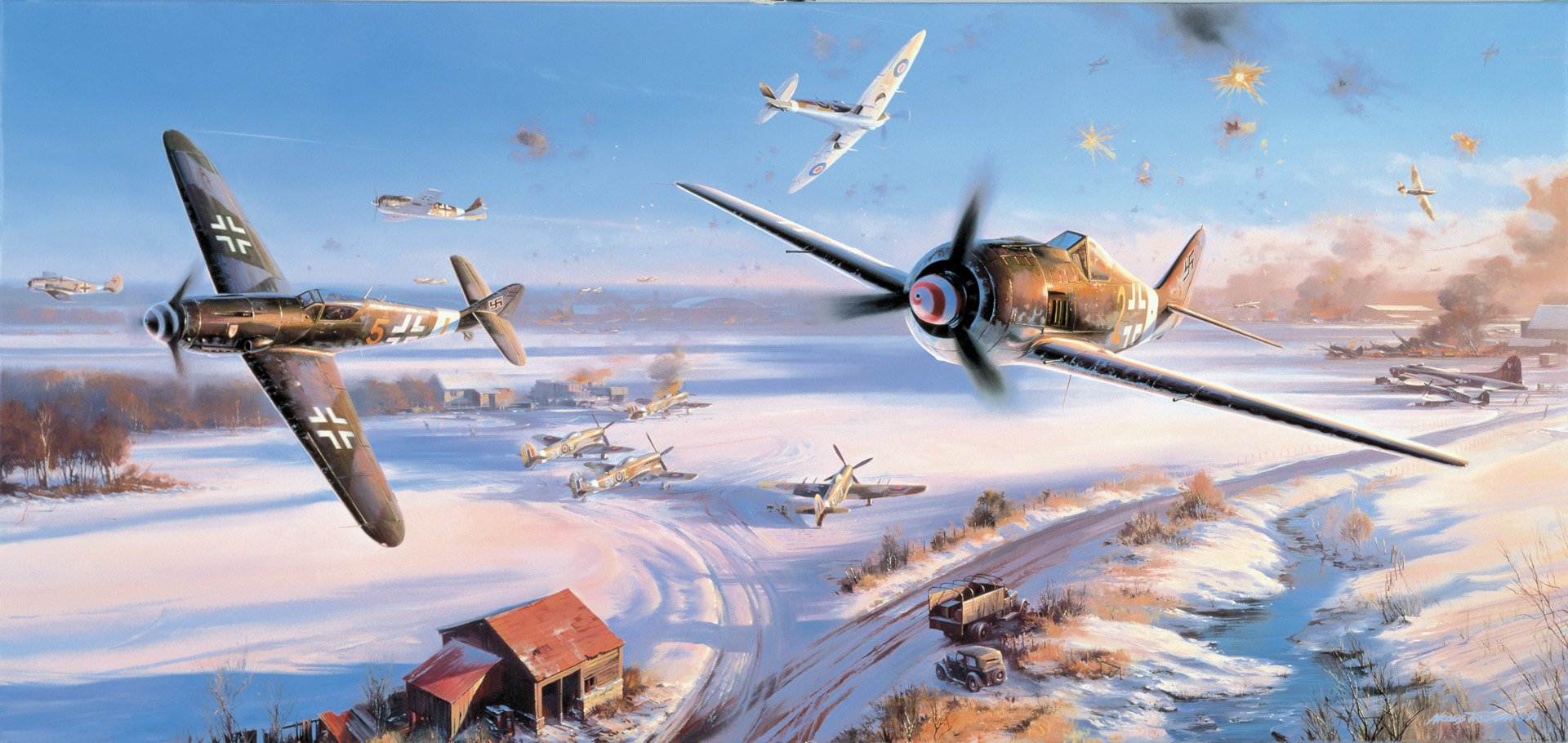This detailed illustration, reminiscent of a painting set in an earlier time, depicts an intense World War air battle over a snow-covered landscape. The sky, a clear blue, is filled with fighter planes of various types, including black planes emblazoned with cross insignia and white aircraft, suggesting an enemy confrontation. In the foreground, some vintage airplanes, detailed with propellers, back wings, and front wings, are in sharp focus, revealing pilots inside, while more faintly rendered planes appear in the deep background. The aftermath of a bombing is evident with several orange balls of light indicating explosions and numerous smoky billows rising from bombed-out buildings below, lending a rusty hue to the scene. The terrain below features a mixture of structures, including a red-roofed wooden barn, cabins, and several old vehicles like a jeep and an army truck with open sides and no roof, likely used for wartime transport. The snow-covered ground, dotted with distant trees and highlighted by the ditch on the right, adds to the somber winter setting of the chaotic air raid.